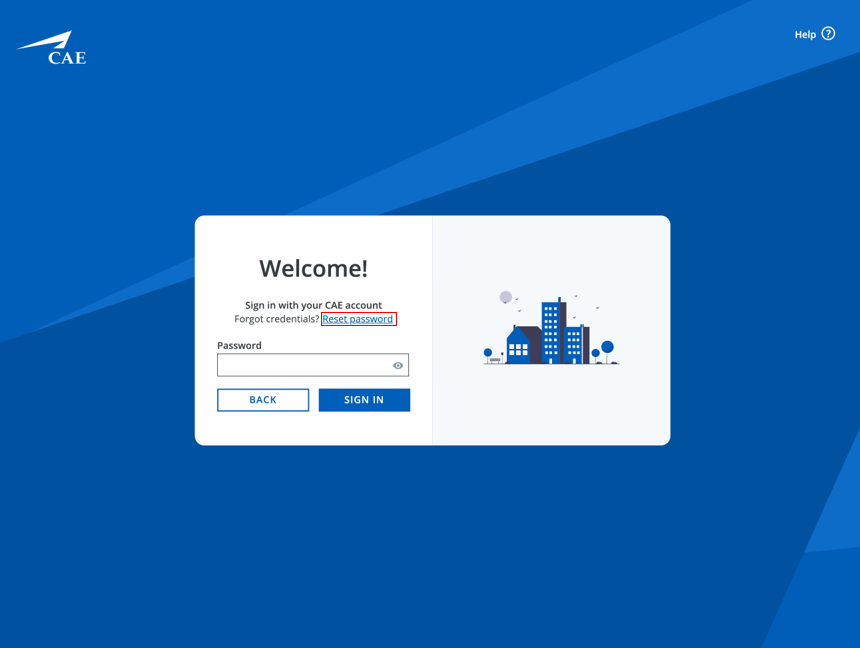In the top left corner of the image, there's a label with a light blue background that reads "Texas." The top right corner displays the word "Help" inside a circular icon with a question mark. The center of the image features a prominent white box with rounded edges, which contains the text "Welcome to Texas." Below this, there is a form for signing in with a CAE account, including options for "Forgot credentials" and fields to enter a password. The password field is highlighted in red, with an eye icon next to it for toggling visibility. To the right of these fields, there is a blue button labeled "Back," and a darker button labeled "Sign In." The background includes a scenic illustration of a house, a tall skyscraper, and multiple small trees, creating a vibrant and welcoming atmosphere. Additionally, a hot air balloon can be seen floating in the background, adding to the lively setting, signifying that this is a login page for a CAE account.